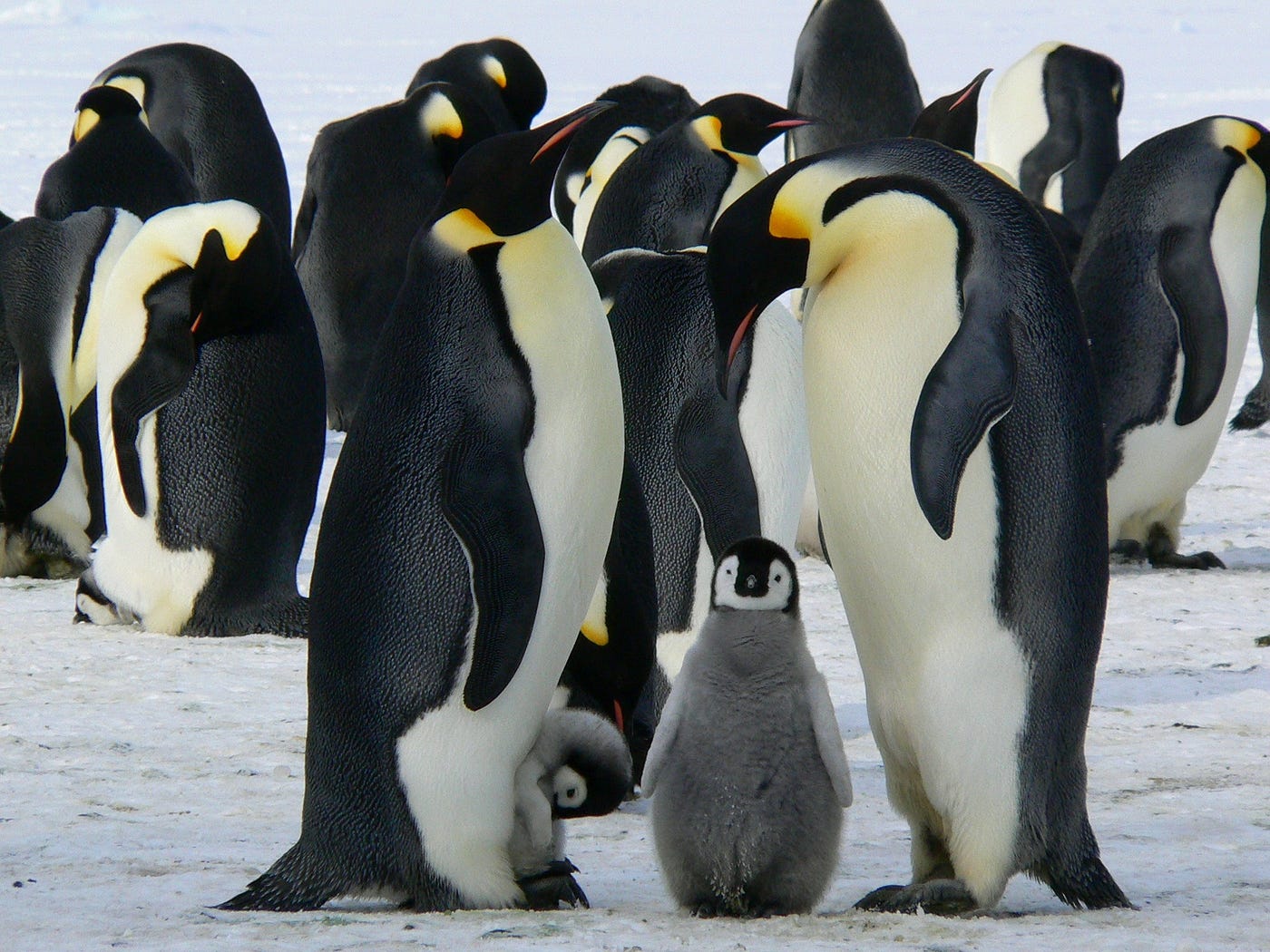This image captures a lively group of approximately 12 to 13 penguins gathered on an icy, snowy surface. The penguins, with their distinctive black-and-white markings and splashes of orange and yellow near their temples, resemble guests in tuxedos at a social gathering. Most of the penguins are large adults standing upright, exuding a sense of regality. Among them, a notable fluffy young penguin with gray fuzz stands out, positioned centrally and looking directly at the viewer. This young penguin is flanked by two attentive adult penguins. Additionally, there is another baby penguin nestled closely into the side of one of the adult penguins, with its little head partially obscured by black fuzz. The background reveals another cluster of adult penguins standing, some in pairs, against a backdrop of white sky and slightly dirty ice, tinged with yellowish pollution. The icy ground is also marred with spots of black and brown. The overall scene is enchanting, capturing a moment of communal warmth amid the stark, frozen landscape.